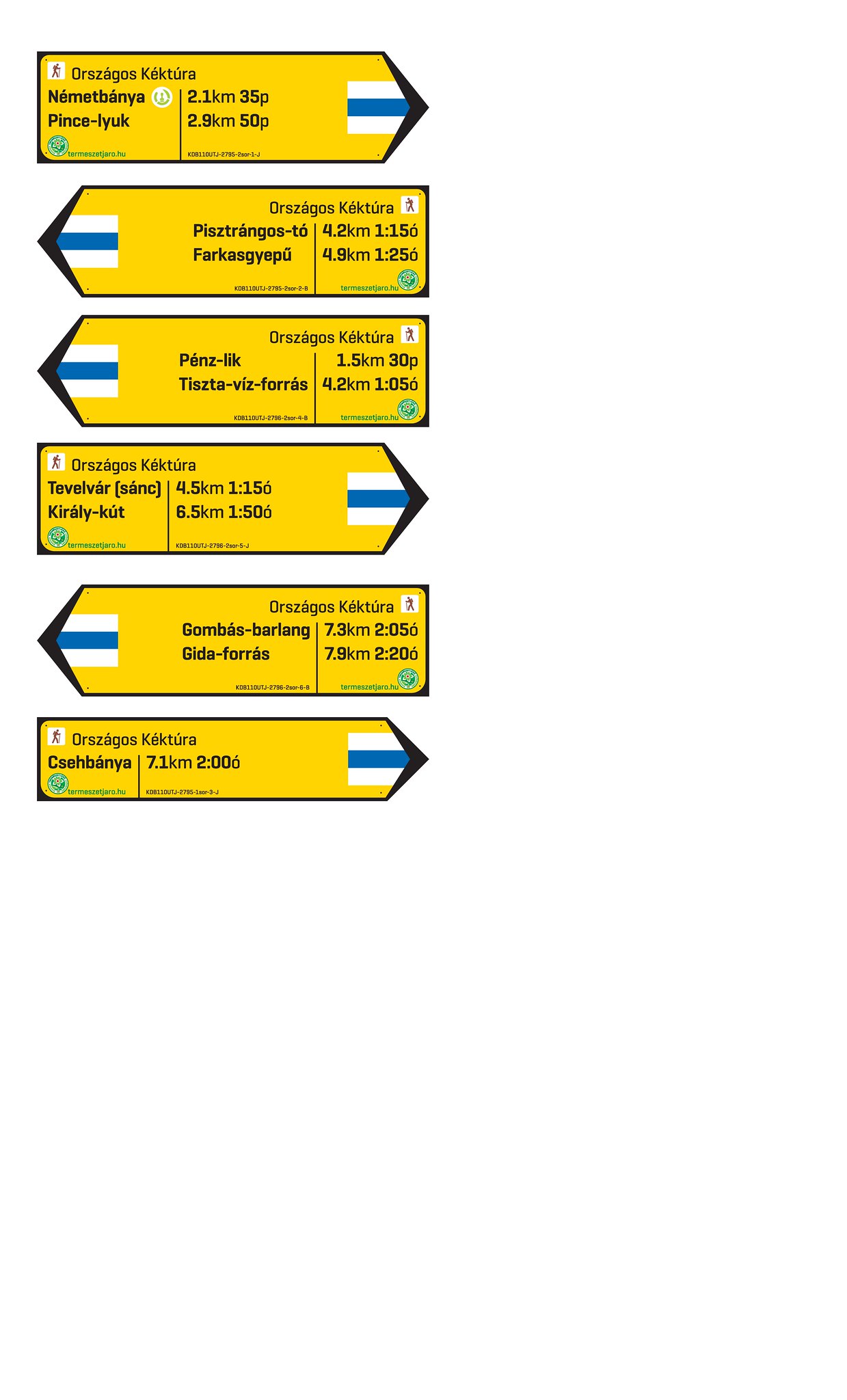The image depicts several bright yellow directional signs, each adorned with a black border, and vividly pointing in various directions. These signs, resembling oversized post-it notes, indicate distances in kilometers to different locations. Each sign features a small pedestrian symbol at the very top left corner. The yellow arrows alternate directions—some pointing right, others left—and each one displays two location names accompanied by their respective distances. The distances are presented in a foreign language, with figures such as "2.5 KM 35P" and "4.2 KM 15P" being visible. These arrows provide essential navigational information for pedestrians, guiding them to various destinations. They are set against a white background for clear visibility.